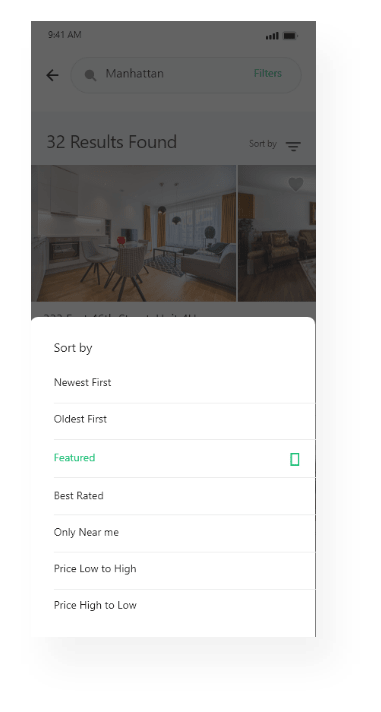A phone screenshot depicting a search for places in Manhattan. The background is darkened, creating a subdued backdrop for the primary focus: a prominent pop-up window occupying about half of the screen. This white window, titled "Sort By," presents a series of sorting options including Newest First, Oldest First, Featured, Best Rated, Only Near Me, Price Low to High, and Price High to Low, indicating it's a filter tool for browsing listings. Above this pop-up, the standard phone interface elements are visible: the current time in the top left and service bars along with battery level in the top right. Below the pop-up, the website or app's search bar displays "Manhattan," confirming the search criteria. The results section beneath the search bar shows "32 results found" with a drop-down arrow that leads to the sort-by menu, emphasizing the context of the filter. Detailed images of the listed properties are partially visible at the bottom, hinting at a variety of homes or apartments available in Manhattan.